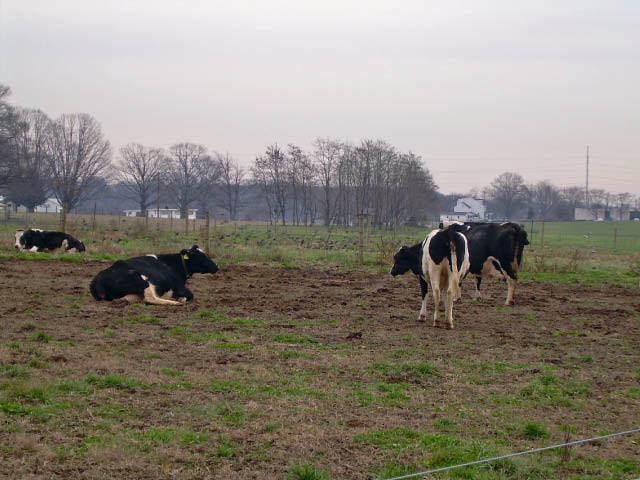In this evocative farm scene, four cows occupy the center of a field surrounded by a sparse, wintry landscape. The predominantly black and white cows are scattered about; two are on the left side of the image, with one lying down and the other standing, while two more are positioned to the right, displaying their hindquarters as they wander and graze in a muddy grass patch. The cold, gray sky casts a subdued light over the area, reflecting a barren winter ambiance. In the background, several leafless trees stand starkly, their branches lifeless and brown. Adding to the pastoral setting, four white buildings—likely farm structures—are visible, with a distant fence enclosing the area, indicating that this is indeed a farm. A utility post with power lines can also be seen to the right, enhancing the rural backdrop. There are no people or other animals in sight; the cows placidly dominate this quiet, cold winter day's landscape.